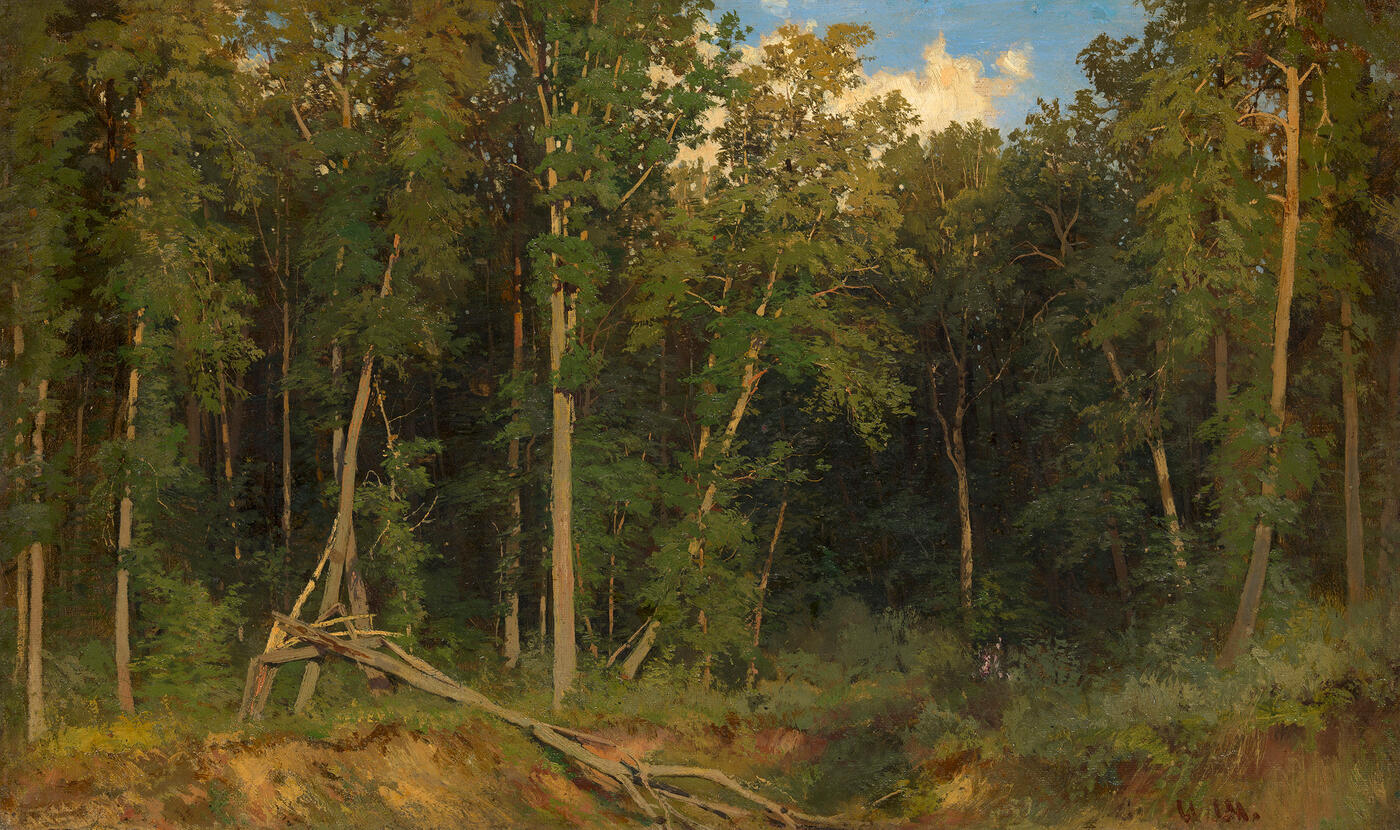In this detailed painting of a forest scene, a realistic depiction captures a vibrant woodland under a bright blue sky dotted with puffy white clouds. Dominating the landscape are tall, thin trees with green leaves starting about a third of the way up their trunks and extending to their leafy treetops. There is a noticeable absence of pine trees. The ground level is rich with life, featuring an abundance of grass, small shrubs, and undergrowth. Toward the left side, the scenery includes a dirt incline that appears scraped, revealing more of the brown earth, with a fallen tree trunk bending down into a valley between two inclines. Meanwhile, the right side of the ground is covered more densely with vegetation. A striking element of the scene is a broken tree trunk on the left side, adding a sense of natural drama to the portrait. This art piece vividly portrays the complexity and beauty of the forest, making the viewer feel as if they are standing within a pristine and serene natural environment.